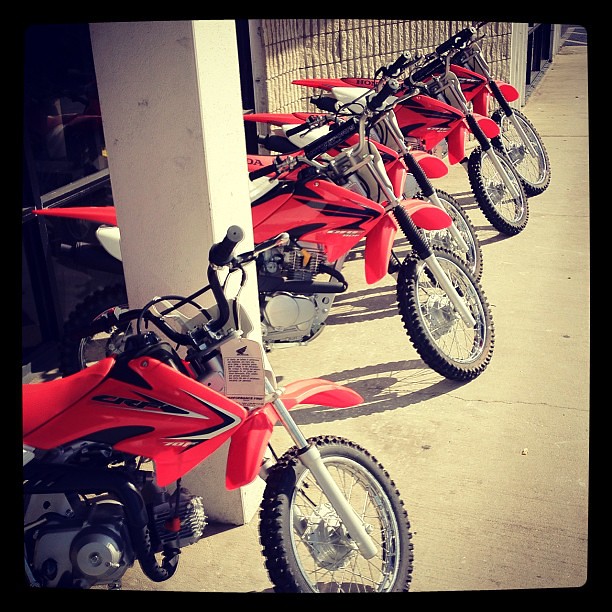This color photograph captures the front of a motorcycle dealership. Prominently displayed are five identical red dirt bikes with knobby front tires, white forks, and distinctive red fenders. Next to the handlebars, there's a flared red piece, adding to their sleek design. These are not bicycles but motorized dirt bikes, all parked neatly in a row on a broad concrete walkway in front of the building. The one in the foreground, positioned just before a large white post, draws immediate attention. The bikes feature tags, likely price tags, and the thick black tires with wire spokes suggest their ruggedness. The dealership’s exterior includes a plate glass window or door to the left and a concrete wall with a narrow rectangular pattern to the upper right. The setting appears well-organized and ready for potential buyers.